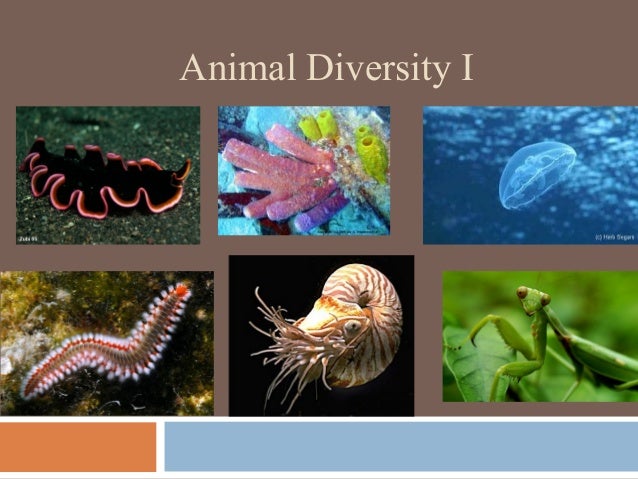The image features a grid of six smaller photographs, set against a dark gray background with light tan text at the top that reads "Animal Diversity I." The grid is composed of two rows of three images each. 

In the top-left corner, there is a photograph of an unidentifiable black sea creature with wavy, white-edged sides. To its right, in the middle of the top row, is an image of colorful sea coral, with pink and yellow hues. The rightmost image in the top row showcases a jellyfish floating in blue water, with its bell-shaped body prominently displayed.

Moving to the bottom row, the leftmost image presents a unique fuzzy sea creature, displaying a white hairy outline against its greenish body. The center image features a nautilus, its white shell adorned with reddish-pink lines and an eye visible among its extended tendrils. The final image on the bottom row, to the right, is a close-up of a green praying mantis resting on a leaf.

The overall scene is bordered partially by orange at the bottom and extended light blue on the lower part, bringing a vibrant contrast to the natural subjects captured within the six photographs.